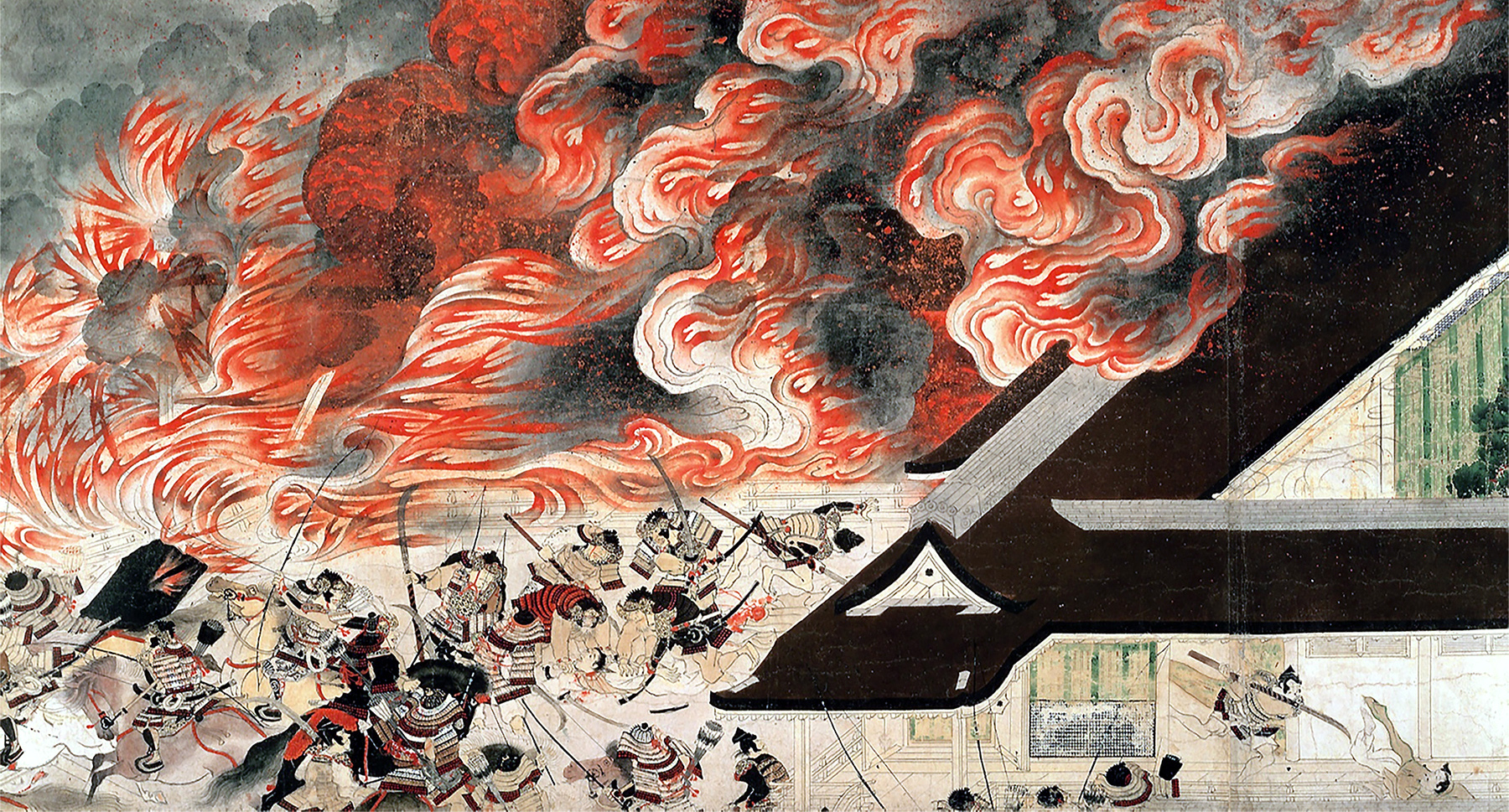This is an image of an ancient Japanese painting depicting a dramatic battle scene. Spanning from the left to the right, the sky is engulfed in flames rendered in vibrant orange with dynamic white streaks, complemented by billowing black and gray smoke in the upper left corner. In the lower left-hand part of the painting, several armored soldiers are visible, some drawing longbows while others wield swords. Among them, one soldier is mounted on a horse. The ground beneath them is a unique yellowish-pink hue. The right side of the image shows part of a building with a shallow hall, where chaos continues as soldiers storm in. One soldier appears to have penetrated the building and is poised to stab an opponent who has fallen to the ground inside. The flames and smoke extend above the building, creating a sense of urgency and chaos that dominates the upper portion of the painting. The colors used are red, black, yellow, gray, and off-white, illustrating the intensity of the battle.